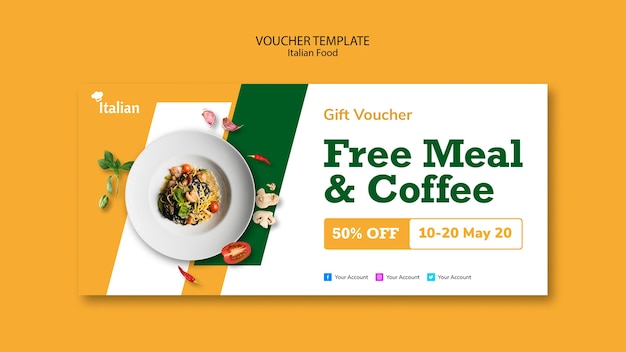This is a detailed picture of an Italian food gift voucher template with a vibrant yellow background. Centrally, the voucher prominently features a dish of Italian food, possibly pasta adorned with vegetables and shrimp, surrounded by basil, tomatoes, chilies, mushrooms, and garlic. The voucher itself is designed with a stylized Italian flag on the left side, incorporating green, white, and orange stripes. The voucher text is displayed with a mix of green, white, and orange colors. At the top, "Gift Voucher" is written in yellow, followed by "Free Meal and Coffee" in green. Below, two connected boxes display additional offers: the left yellow box with white letters reads "50% off," while the adjacent white box with orange letters notes the date range "10-20 May 2020." Social media icons for Facebook, Twitter, and another platform can be seen at the bottom of the voucher. The overall composition is vibrant and eye-catching, intended to attract customers with its generous offers and appealing design.